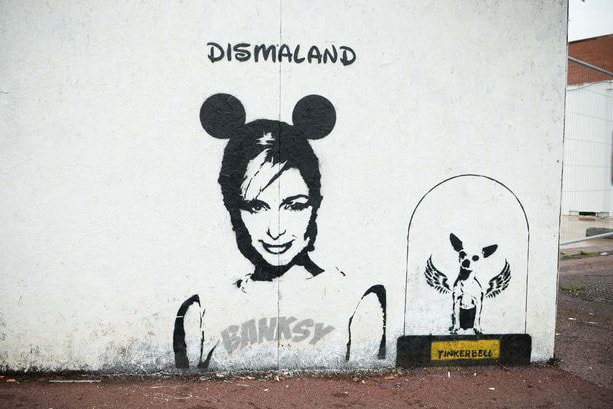This image features a Banksy mural painted on a worn and slightly messy white stucco wall of an older building. The scene is centered around Paris Hilton wearing Mickey Mouse ears, depicted in a white sleeveless shirt with "Banksy" written in gray letters. Above her head, in Disney-style font, is the word "Dismaland," spelled out as D-I-S-M-A-L-A-N-D. To her right, there's a chihuahua with wings inside a glass case, accompanied by a yellow rectangular plaque with "Tinkerbell" written in black letters, also in Disney font. The surroundings include another distant building, a mix of concrete and brick walls, and cigarette butts scattered on the ground.